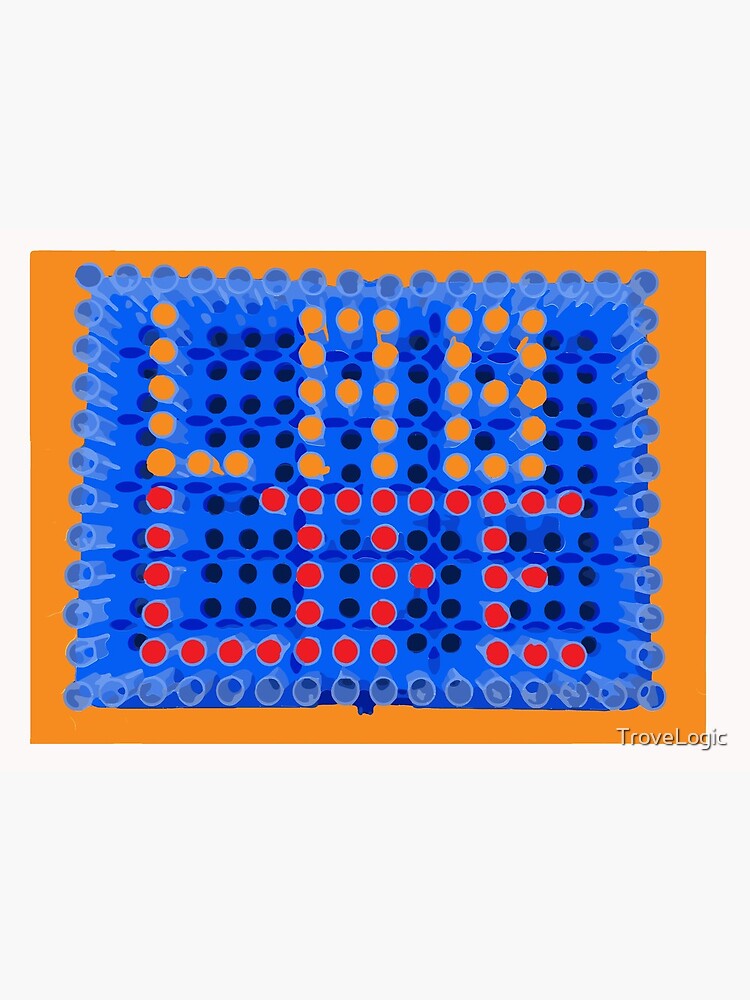This is a landscape-oriented image of what appears to be a grid-based puzzle or game, possibly sourced from a website. The image features a prominent orange border surrounding a grid filled with circular tubes or holes, with many of these holes left unoccupied. The central section of the grid primarily consists of empty spaces and light blue tubes. Along the top border, orange tubes spell out "LAB," while the bottom border is populated with reddish tubes forming the word "LIFE." In the lower right-hand corner of the image, the word "TrovaLogic" is written in white text. The overall design appears to be a compact three-by-three structure, with the filled-in parts potentially forming the number "614." The absence of additional identifying information suggests it could be part of an interactive puzzle or game meant for problem-solving.